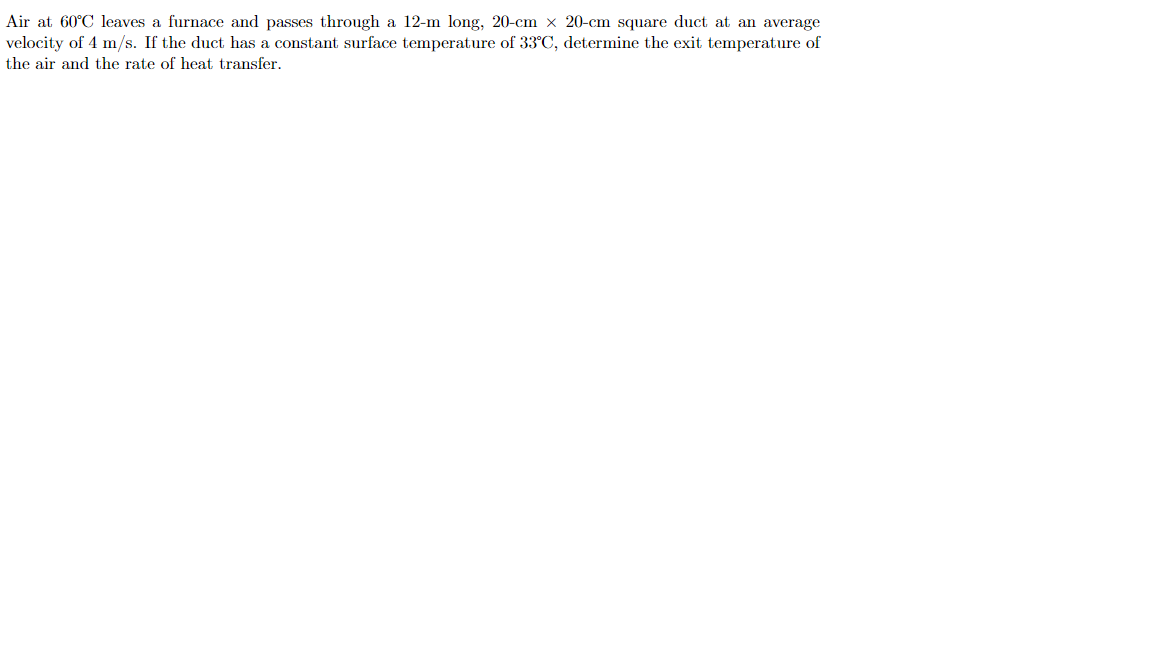The web page displays a minimalistic design, featuring a plain white background with a single block of black text. The text, focused on a thermal dynamics problem, reads: "Air at 60 degrees Celsius leaves a furnace and passes through a 20-meter long, 20-centimeter by 20-centimeter square duct at an average velocity of 4 meters per second. If the duct has a constant surface temperature of 33 degrees Celsius, determine the exit temperature of the air and the rate of heat transfer." The page is devoid of any additional elements, graphics, or information.